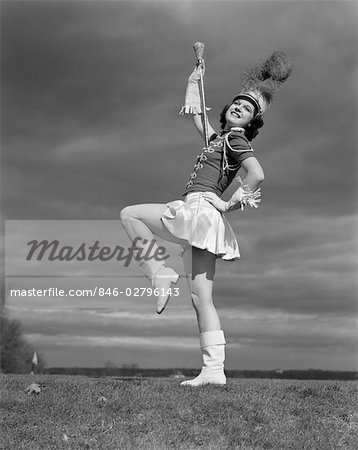In this black and white photograph, a light-skinned woman is performing a marching band-type dance in an open grassy field. The setting is outdoors, under a cloudy sky with scattered trees visible in the distance. Positioned centrally in the image, she wears a striking costume consisting of a short white skirt, white boots, and white gloves. Her top is darker and tight-fitting. Her dark hair is adorned with a distinctive hat, featuring a white base and a darker feather protruding from the top. In her right hand, she holds a baton or wand, while her left hand rests on her hip, with her left leg raised in an action pose. There is a watermark reading "Masterphile" towards the middle to the right of the image, and text at the bottom left corner providing the address "masterphile.com." The image captures a dynamic moment, highlighting the contrast between her detailed attire and the serene, shaded landscape.